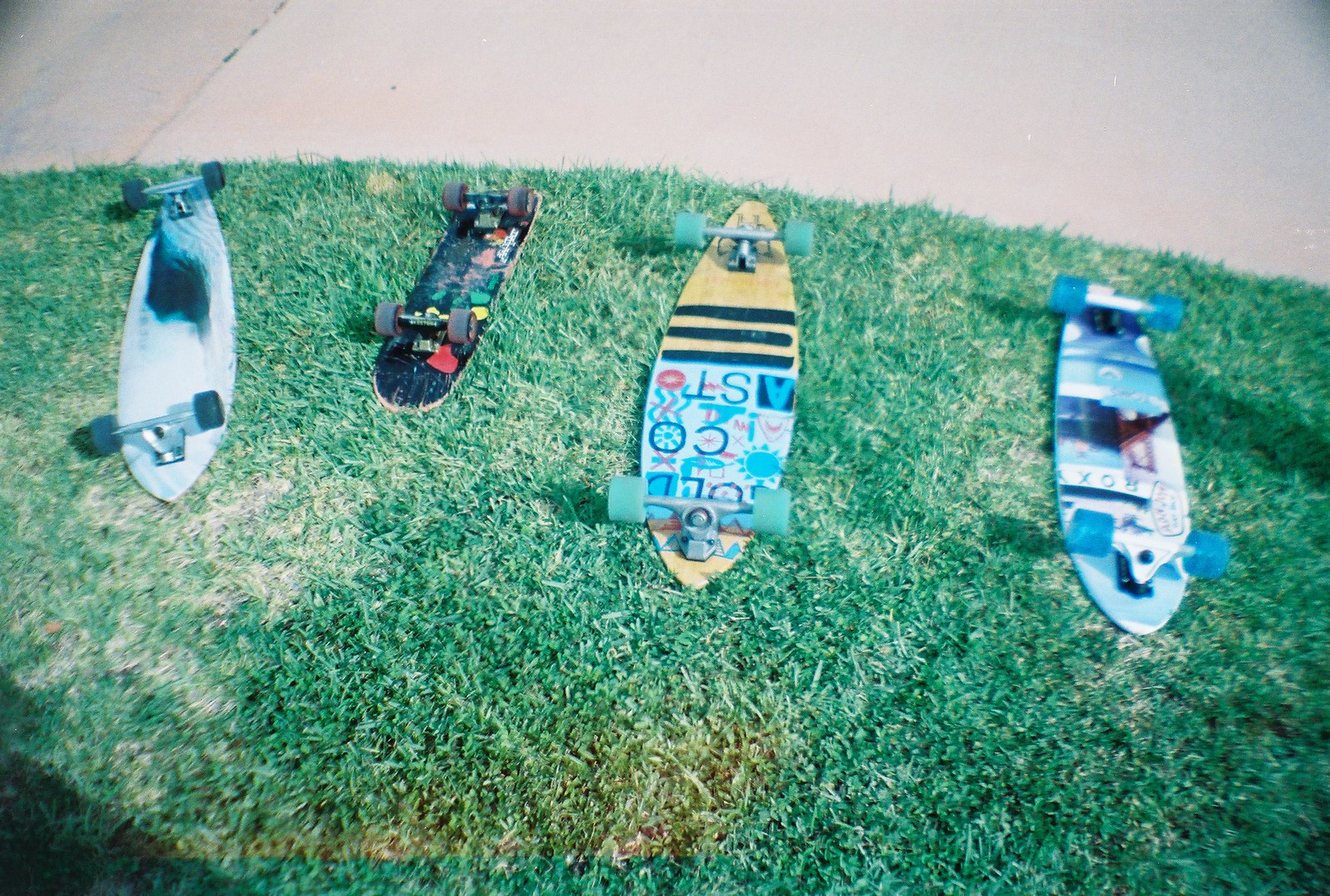The photo is a slightly blurry, overexposed snapshot taken in glaring bright light, depicting four skateboards lying upside down on a neatly mown, bluish green lawn, with the bottom two-thirds covered in grass. The grass includes a small patch of dead grass on the left and a yellowish stain at the bottom center. The top third of the image shows a concrete sidewalk with a visible expansion crack on the left. 

The skateboards vary in size and are arranged with their wheels up. The skateboard on the left has a blurry, black and white deck with black wheels. The next skateboard features a black deck adorned with patches of pink, red, and green, and dark wheels, and is the smallest of the four. The third skateboard has a wooden deck with unreadable upside-down text, light green or blue wheels, and black stripes, resembling a longboard. The skateboard on the right is very blurry but has blue wheels with a blue, black, and white deck design.